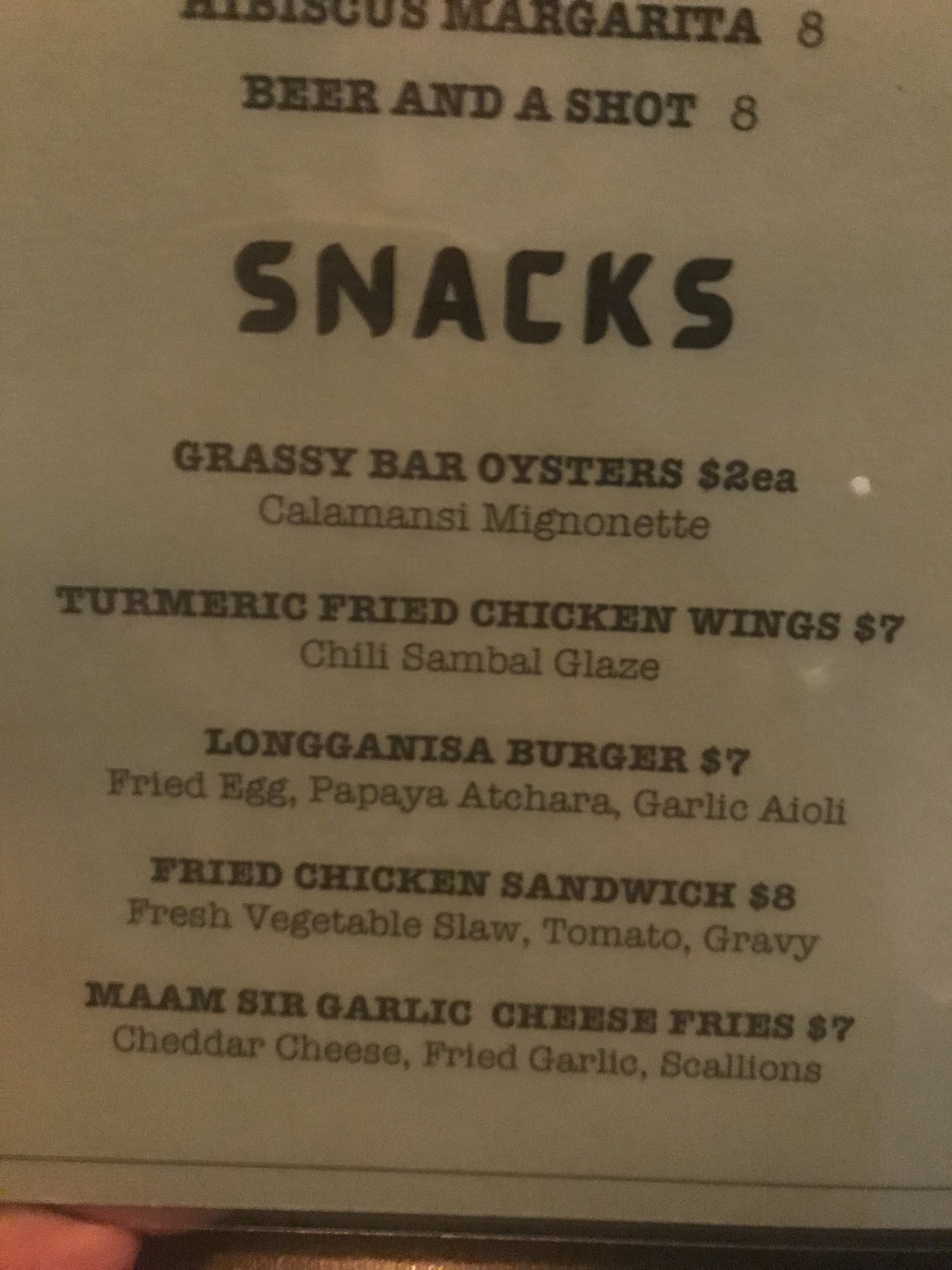A close-up image of a printed menu, primarily showcasing a list of snacks and beverages available at a bar. The top portion of the menu features the partially cropped title "Hibiscus Margarita" with a price of $8. Below it, the menu lists a "Beer and a Shot" also priced at $8.

Prominently displayed in bold letters, the word "Snacks" heads a list of delectable items:
- **Grassy Bar Oysters** - $2 each, with a description of "Calamansi Mignon" in less bold text underneath.
- **Turmeric Fried Chicken Wings** - $7, accompanied by a "Chili Sambal Glaze."
- **Longanisa Burger** - $7, detailed with "Fried Egg, Papaya Atkara, Garlic Aioli."
- **Fried Chicken Sandwich** - $8, featuring "Fresh Vegetable Slaw, Tomato, Gravy."
- **Mam Sir Garlic Cheese Fries** - $7, topped with "Burger Cheese, Fried Garlics, and Scallions."

A hand, possibly the customer's, is visible at the side of the frame, holding the menu for the camera, capturing the rustic charm and diverse offerings of the bar's munchies and drinks.